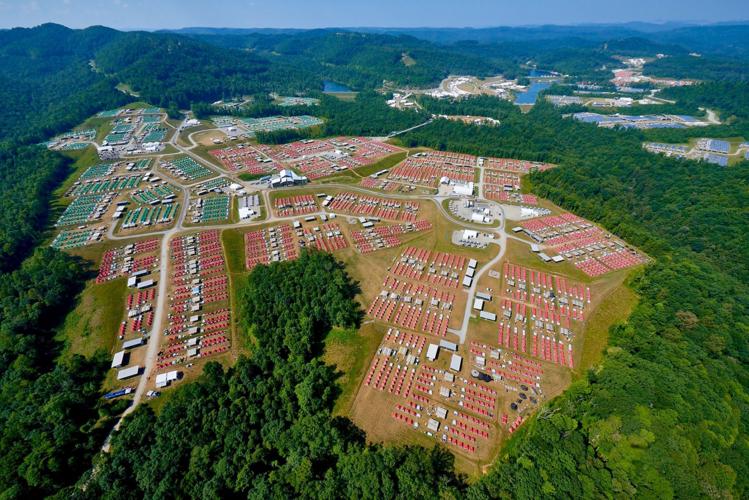This aerial photograph, likely taken by a drone or possibly from a helicopter or plane, captures a sprawling, possibly military base or barracks, enveloped by a vast tropical forest. The developed area is intricately divided into distinct sections, connected by cement roads forming circular patterns. In the heart of the image, a multitude of small buildings, characterized by their red roofs or containers, contrasts against patches of greenery and larger white-roofed structures. To the top right of the image, blue-roofed buildings are visible, while to the top left, a cluster of green-roofed buildings can be seen. The entire base is tightly surrounded by dense forest, with tree-covered hills and occasional rivers stretching beyond the boundaries of the development. The juxtaposition of the orderly, colorful roofs and the lush, encircling forest creates a striking visual of human development nestled within untouched nature.